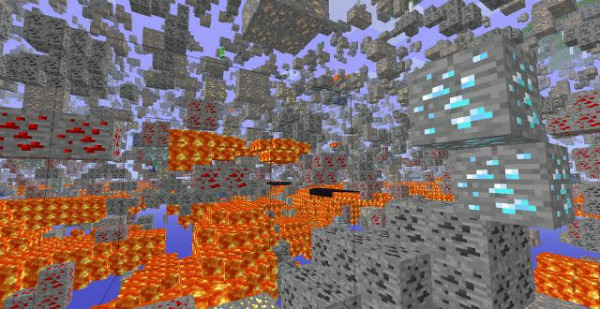The image resembles a cartoon-like or graphic design scene reminiscent of a Minecraft screenshot, featuring a mass of colorful cubes and squares. The background reveals a gradient sky transitioning from purplish-blue at the top to dark blue near the middle, with faint white clouds visible. Gray squares dominate the upper portion, while the lower region hosts a variety of colors. 

At the center and bottom, oranges and rust-colored cubes create a striking contrast, reminiscent of lava. Scattered across the scene are notable details like gray squares accented with red dots, two large squares with bluish dots in the upper right, and a mix of gray and black squares in the bottom middle. Smaller orange boxes are interspersed throughout, especially towards the bottom-right. Different sizes and positions of these squares suggest a pixelated, video game aesthetic, with nearer blocks appearing larger and more detailed.